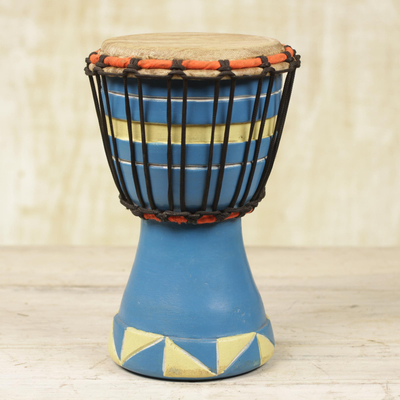The image is a detailed and realistic photo of an African hand drum resting on a light-colored wooden surface. The background features a light tan, draped wall that is out of focus, emphasizing the drum in the foreground. The drum itself has a cylindrical blue base approximately one foot tall, which tapers inward before expanding into a wider cylindrical drum body.

The base of the drum is adorned with alternating blue and white triangles forming a border. Above this, the body of the drum continues its blue coloration, segmented by a pattern of thin and thick white lines. The drum head is made of tan leather, tightly secured by black straps that connect to an orange cord, which runs both at the top and bottom of the drum, ensuring the drum skin's tightness and integrity. This aesthetic combination of colors and patterns, along with its distinct shape, reflects the traditional design elements of African drums.